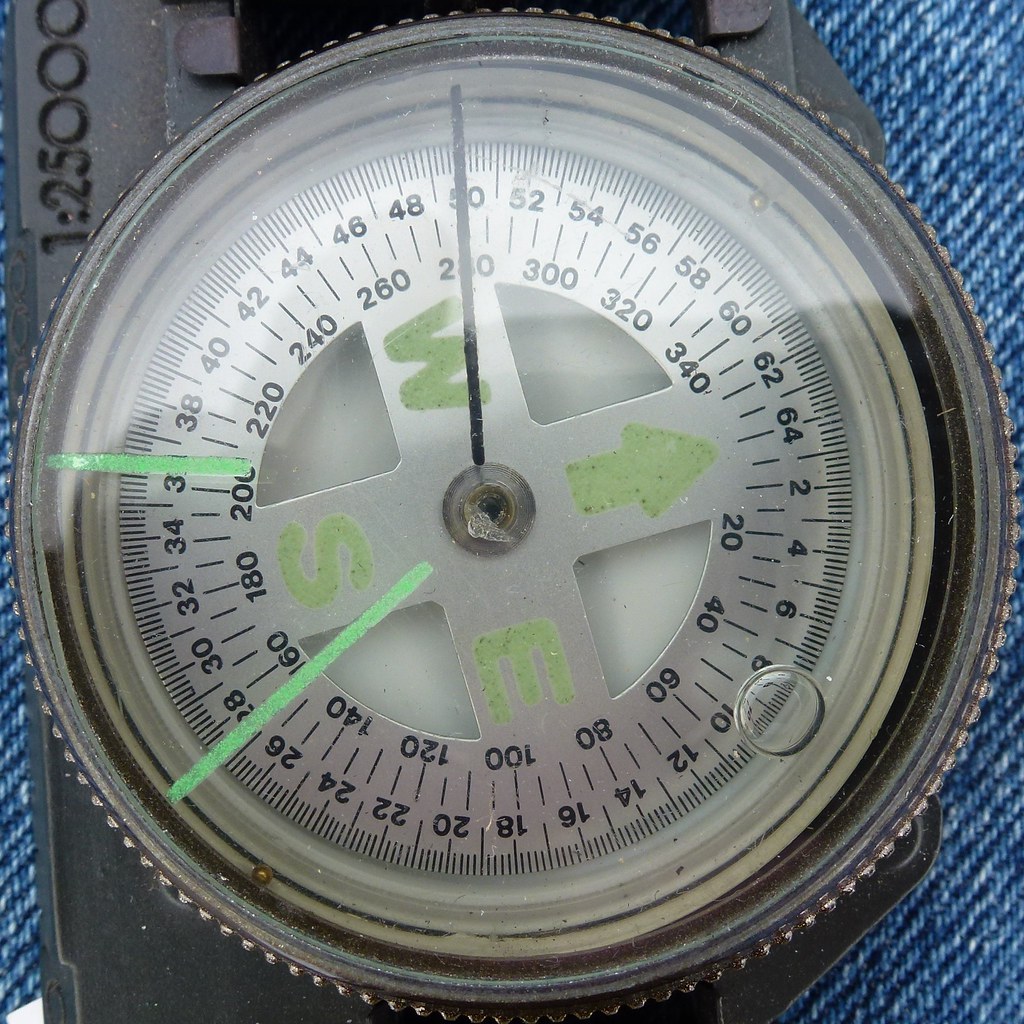A close-up square image prominently features what appears to be a complex instrument combining elements of a compass and a metering device, potentially for a camera. The focal point is a circular, gray compass-like tool with a jagged, knurled edge, filling most of the photograph. The compass face is oriented with North pointing to the right, and labeled in green with the letters N, W, E, and S. Surrounding the compass are two sets of numbers; the outer set ranges from 2 to 64, and the inner set from 20 to 340 degrees, resembling ruler measurement points. Attached to a dark gray metal object that extends from the top to the bottom of the image, the instrument’s background seems to be a blue fabric, possibly denim, interspersed with occasional white threads. Immediately behind the compass, there is a vertical black plastic strip with the engraving "1:25,000," adding to the instrument’s intricate design. The combination of features suggests its use in precise directional and metering measurements.